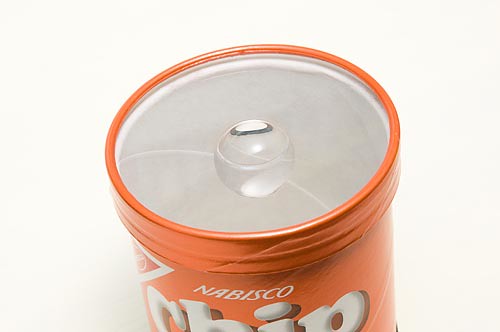A highly detailed image depicts the top view of a cylindrical container, similar to the design of a Pringles can, which houses potato chips. The can itself is vibrant orange in color and occupies much of the background. The primary focus of the photograph is the container's lid, which is transparent and designed with a clear, centrally positioned round or oval knob that appears to screw on. The branding on the container is prominently visible; the word "Nabisco" is printed in white, complemented by a distinctive white triangle jutting out from the left side. Below "Nabisco," the word "Chip" is displayed in a larger font, also in white but accented with gray shadowing, adding depth to the text. The image creates a striking visual focus on the clear lid and branding elements, capturing the essence of the product in a crisp, detailed manner.